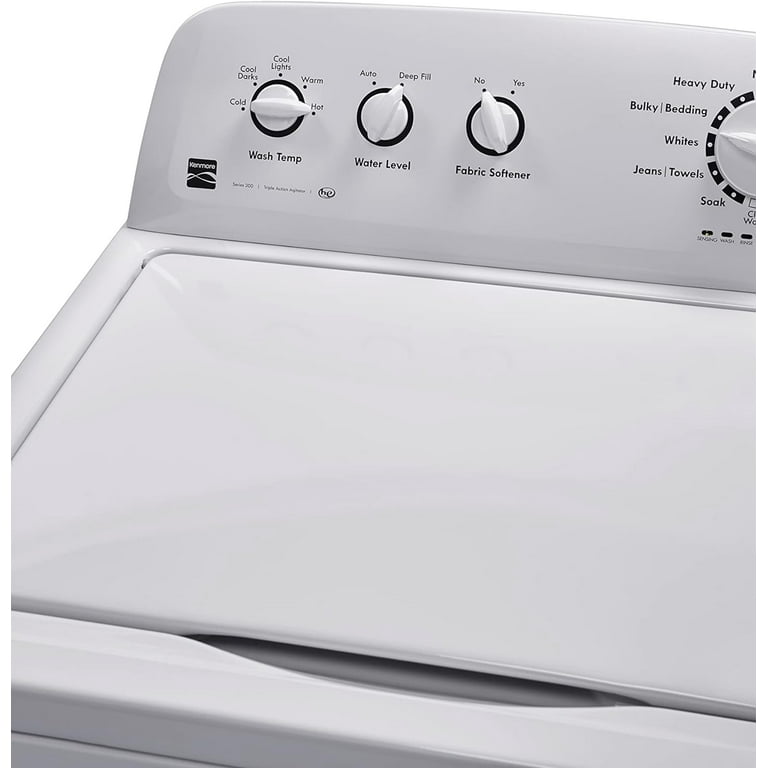This is an image of a high efficiency, white Kenmore washing machine. The machine prominently features the Kenmore logo in black at the bottom left. The top of the washing machine is displayed clearly, showcasing various control dials and settings, despite part of the image being cut off. On the left side, there are three white knobs with black borders. The first knob is labeled "wash temp," which offers multiple temperature settings including cold, cool darks, cool lights, warm, and hot. The second knob is for "water level," with options such as auto and deep fill. The third knob controls the usage of fabric softener, providing simple yes or no options. Additionally, there are settings for different types of loads like heavy duty, bulky bedding, whites, jeans, and towels. The machine has a clean, modern appearance, with a well-organized array of buttons and dials to adjust various washing parameters, making it user-friendly and versatile for different laundry needs.